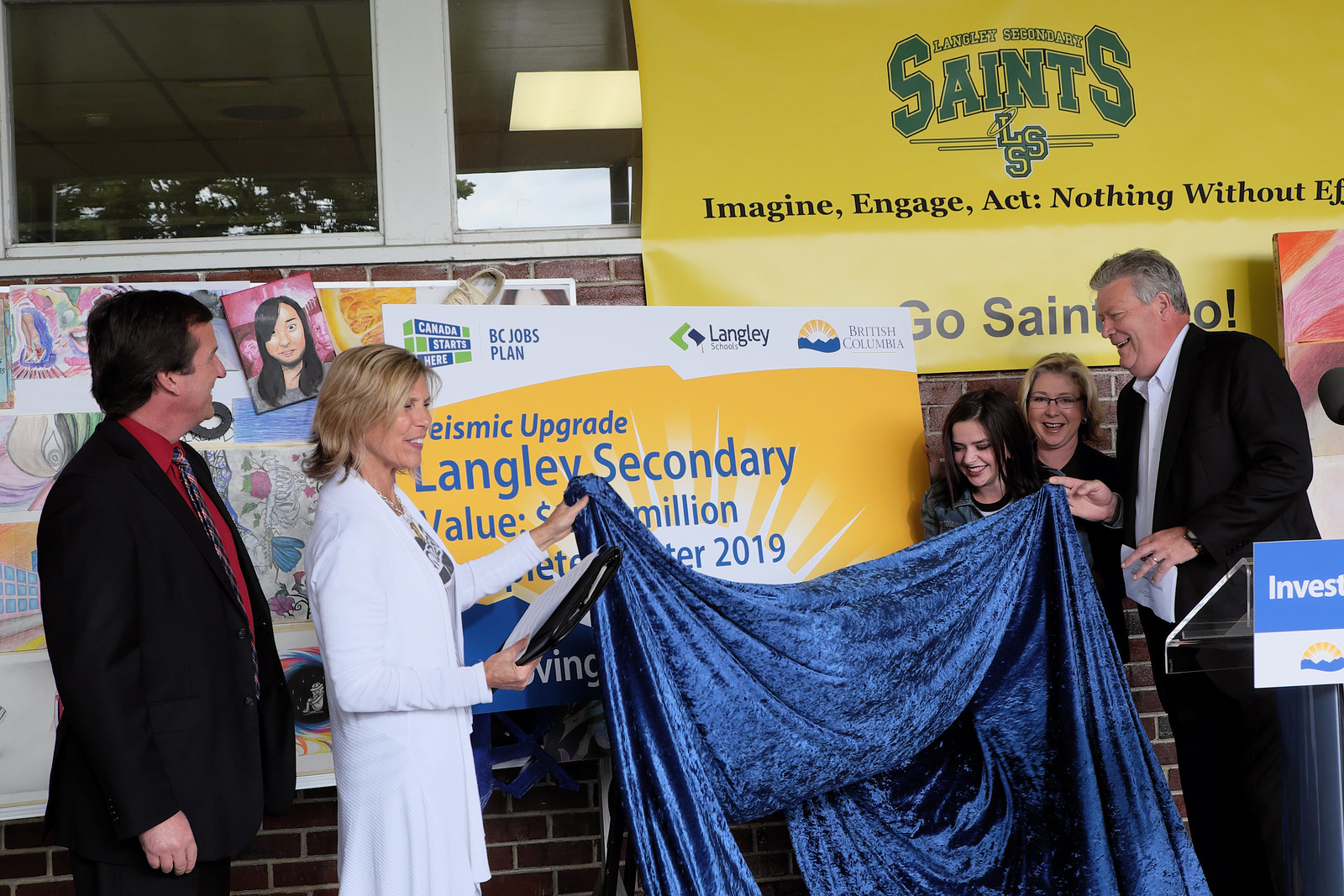In a bustling school hallway adorned with student art, five individuals stand in an unveiling ceremony, holding a blue swath of velvet cloth. The group includes a man in a suit with a red shirt and blue-and-red striped tie on the left, standing beside a woman in a white dress with blonde hair holding a binder. Behind her stands a brunette young woman looking down at the cloth, with a blonde woman smiling behind her. On the far right, an older gentleman in a black blazer with a white button-down shirt holds the other end of the velvet fabric. 

Two prominent banners hang on the wall behind them. The top banner, yellow with the words “Langley Secondary Saints, LSS, Imagine Engage Act” and the slogan "Go Saints Go," suggests school spirit. Below it, an orange banner reads “Canada Starts Here, BC Jobs Plan, Langley Secondary, value something million, 2019, Langley Schools in British Columbia,” highlighting a significant project or upgrade related to the BC Jobs Plan. Among the lively backdrop and community engagement, the scene appears to celebrate a pivotal moment for Langley Schools on a clear day.